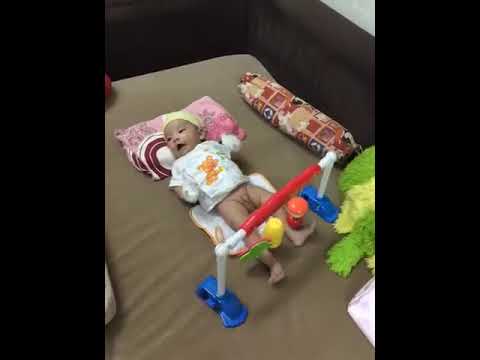This image showcases a baby lying flat on a floor covered in gray tiles, positioned at the center of the small, rectangular horizontal frame. A moderately wide black band flanks either side of the image. The baby is on a blanket, with a pinkish pillow, adorned with a white and red circular design, providing head support. The baby appears awake, wearing a shirt with a bear graphic, and a yellowish cap. Notably, from the waist down, he is nude, indicating a potential diaper change.

Above the baby’s torso, a mobile with three hanging figures, attached to a plastic cross-piece on two feet, is evident. At the baby’s feet lies this engaging plaything. On the right side of the image, a large green and light-green stuffed animal, resembling a frog with discernible front legs, is partly visible. Additionally, the top right corner highlights the presence of a white object, along with a rolled-up blanket that the baby cannot reach. The overall setting suggests a changing platform or bed with a tan mattress, set against a backdrop that includes dark brown couch or chair elements and possible black drapery.